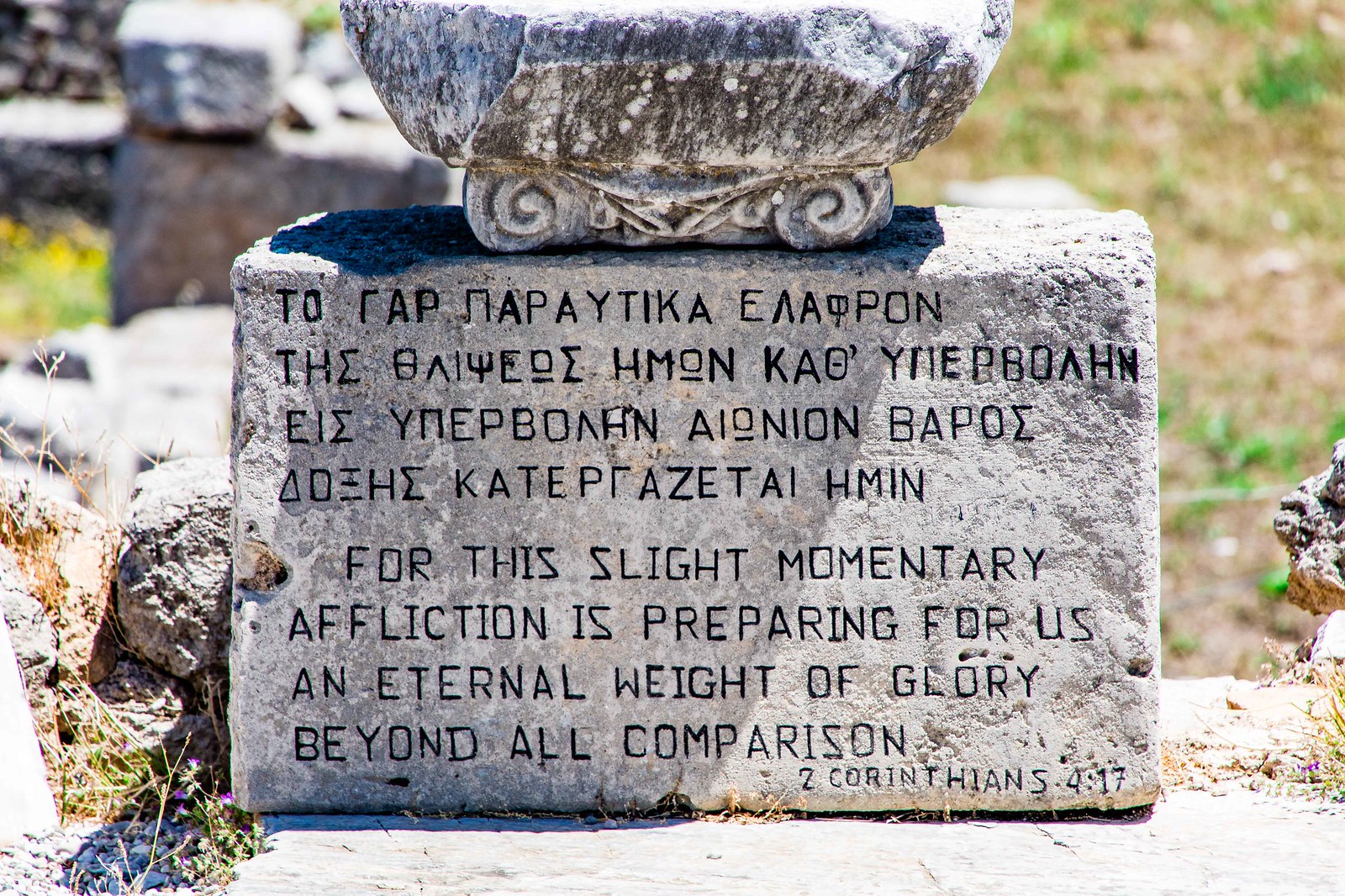In this image, set in an outdoor cemetery under the bright midday sun, the scene prominently features a large memorial tombstone positioned centrally. The ground surrounding the tombstone is mostly grassy, with patches of both green and brown, indicative of early spring or fall. The tombstone itself is a grey block stone adorned with a decorative top, which appears to be partly cut off in the photo. The lower portion of the tombstone is embellished with scrollwork, possibly serving as a holder for flowers.

The stone's upper section contains inscriptions in what may be Hebrew, although it’s not entirely clear. Directly beneath this, in block lettering, is a translation of the text: "For this slight momentary affliction is preparing for us an eternal weight of glory beyond all comparison," from 2 Corinthians 4:17. The cemetery setting includes other blurry, out-of-focus tombstones and memorials, more discernible in the upper left corners. The lighting casts shadows downward toward the bottom left, enhancing the visibility of the textures and colors—green, brown, gray, black, yellow, and orange—of the grassy area and memorial stones.